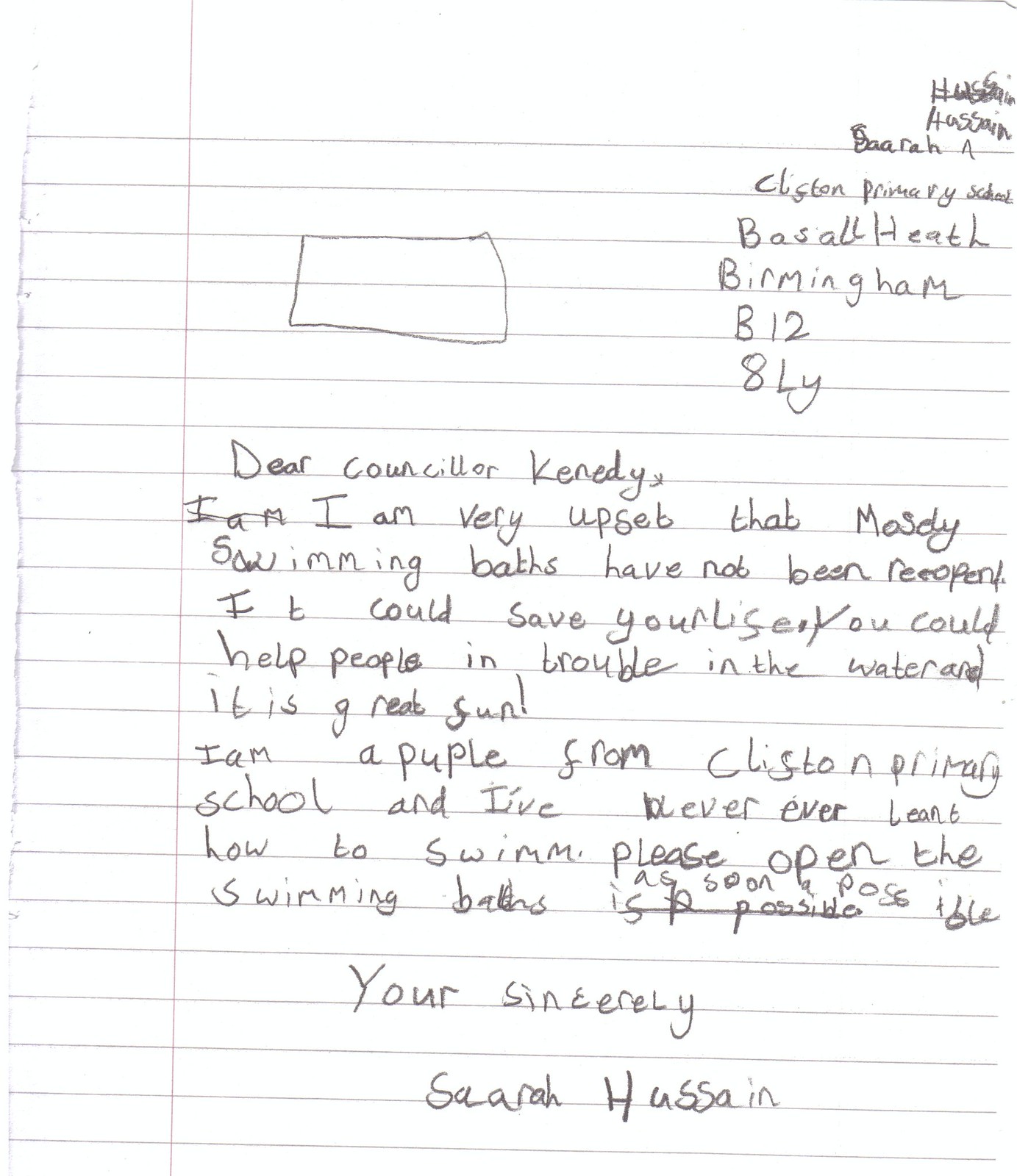This is a photograph of a handwritten note from a child to a school counselor, created on a lined page from a composition notebook. In the upper right corner, there is a printed box containing the child's details: "Basil Heath, Birmingham B12 8LY." The note itself reads:

"Dear Counselor Kennedy,

I am very upset that Mosley Swimming Baths have not been reopened. It could save lives and help people in trouble in the water. I am a pupil from Chilston Primary School and have never learned how to swim. Please open the swimming baths as soon as possible.

Yours sincerely, 
Sarah Hussein."

The handwriting is indicative of a young child, with noticeable spelling errors and a somewhat disorganized layout, emphasizing the heartfelt plea for reopening the local swimming facility.